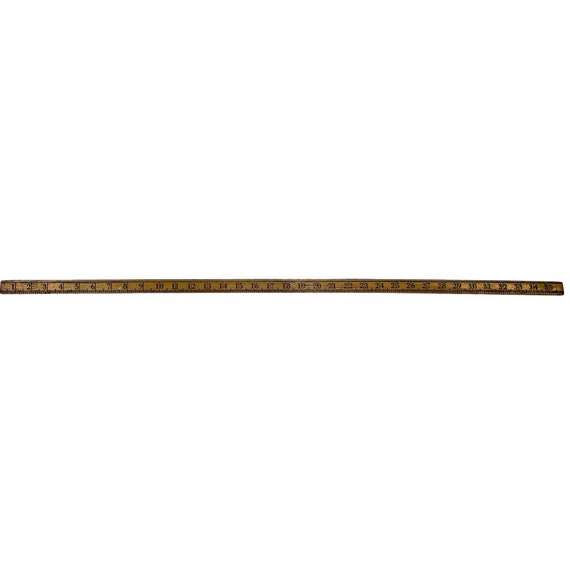The image depicts an antique wooden measuring tape, stretching horizontally from left to right, against a mostly white or transparent background. The tape has a long, thin, yellow-brown stick appearance, lined with black markings and numerals. These numerals, which start at one on the left and incrementally increase, possibly up to 35 or 36, are engraved in dark brown or black. The tape is divided into inch segments with lines marking each number, making it look like a yardstick. The ruler's length spans the entire picture, filling width from edge to edge, and despite its aged appearance, the initial numbers are clearly visible while those towards the end become harder to read due to darkening. The outer edges of the tape are also lined in black.